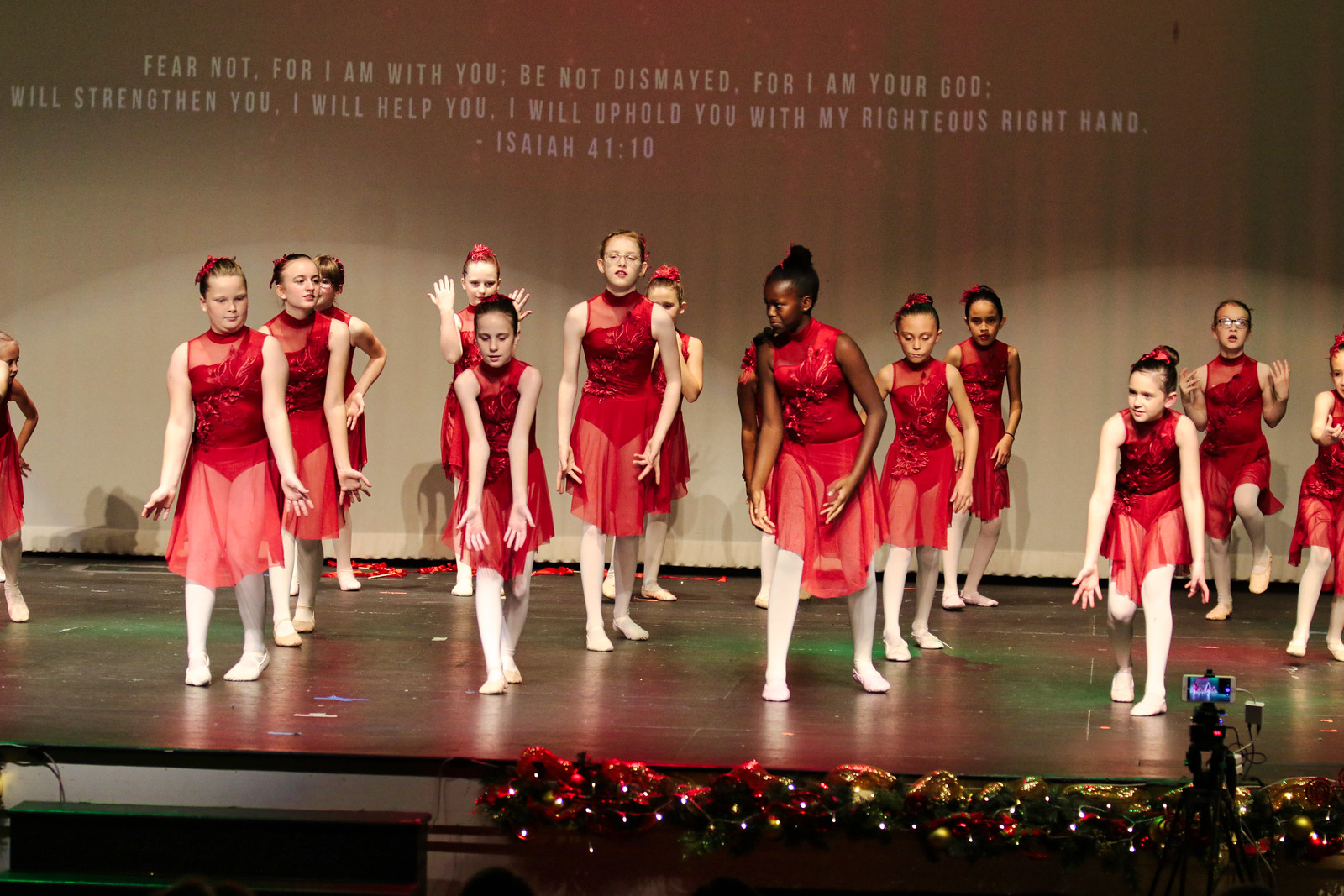On a wooden stage adorned with Christmas lights and garland decorations, a group of young female dancers performs, captured mid-dance step. Each girl, dressed in a red tutu and white ballerina slippers, has her hair elegantly tied up with ribbons. They form several diagonal rows, creating a dynamic, engaging composition. A white curtain serves as the backdrop, on which a powerful message is projected in white text: "Fear not, for I am with you. Be not dismayed, for I am your God. I will strengthen you. I will help you. I will uphold you with my righteous right hand. - Isaiah 41:10." A recording device is visible in the bottom right corner, capturing the enchanting performance illuminated by the festive stage lights.